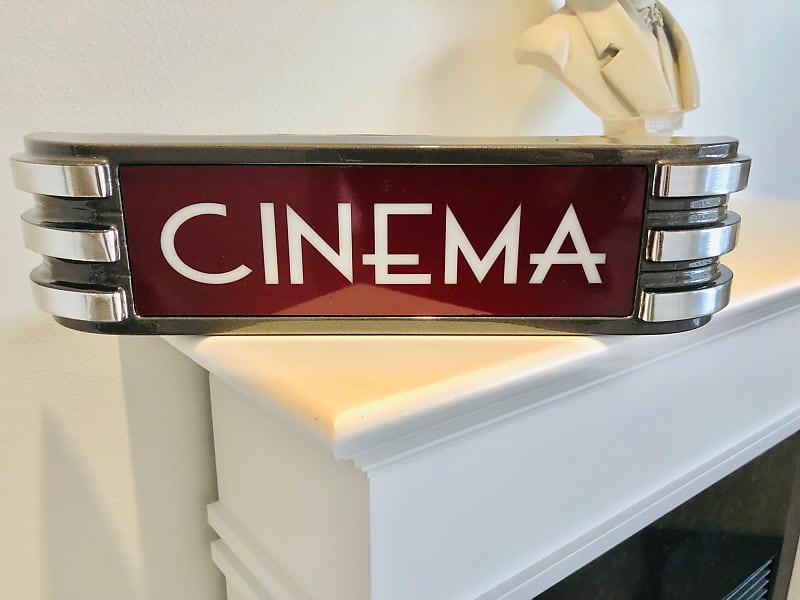The image depicts a vintage cinema sign featuring the word "CINEMA" in white capital letters against a maroon background. The sign is rectangular, bordered on each side by three silver, stripe-like protrusions. The remainder of the sign showcases a sleek, steel-gray finish. Positioned above the sign is a bust sculpture, displaying only the top part of a jacket and what seems to be a necklace, resting atop a pedestal. The entire scene is set upon a white fireplace mantel, which is partially visible at an angle, with a white wall serving as the backdrop.